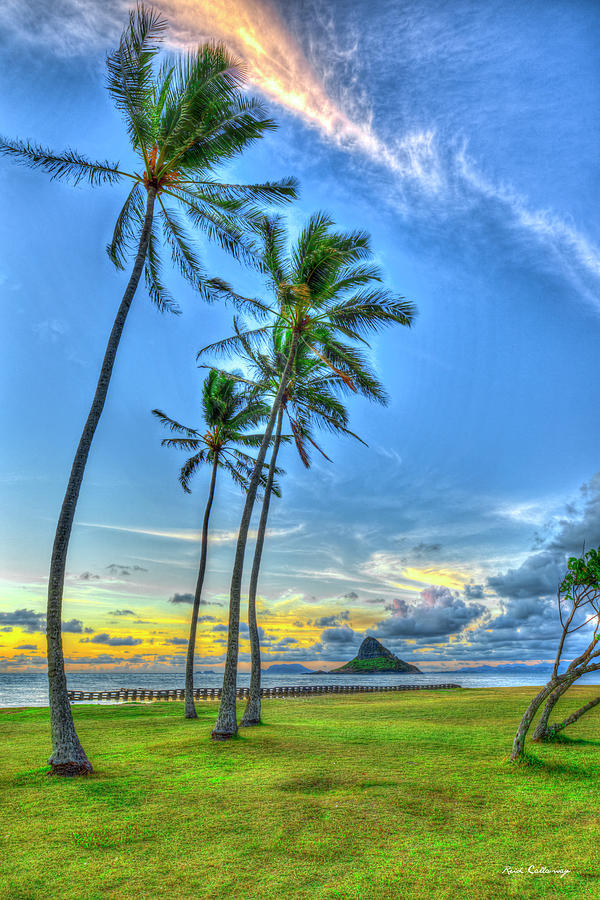In this vibrant and detailed painting, a summertime beach setting unfolds with a lush grassy landscape, unlike a typical sandy shore. Dominating the foreground are three or four towering palm trees, their needle-like leaves clustered at the top, stretching from the base to the top of the image. The pointillism technique used for the grass lends a textured, dotty appearance, adding a unique visual depth. Behind the trees, a wooden fence, or possibly a pier, marks the boundary between land and sea. In the mid-ground, a rocky, potentially volcanic island emerges, giving way to an expansive body of water that extends into the horizon. Further in the distance, another island can be seen. The sky, occupying the top two-thirds of the picture, is a vast canvas of blue, adorned with a stunning sunset that bathes the scene in warm hues of yellow and orange. A fascinating cloud formation, resembling a galaxy or Milky Way, arcs across the sky, enhancing the painting's celestial ambiance. The artist's signature is subtly visible in the bottom right corner, adding a personal touch to this serene and captivating landscape.